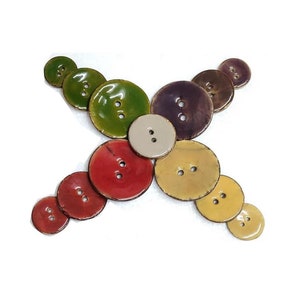The image is a professionally taken photograph showcasing an arrangement of buttons set against a clean, white background. The central element is a medium-sized, glossy, silver-white button with two holes. Radiating from this center button, the buttons are organized into an X shape. Each arm of the X consists of three overlapping buttons: a large button at the base followed by a medium-sized one, and a small one at the tip. The color scheme of the buttons is as follows: the top left features green buttons, the top right has purple buttons, the bottom right displays yellow buttons, and the bottom left includes red buttons. This meticulous arrangement resembles the petals of a flower, with the central silver-white button serving as the focal point. The glossy finish on the buttons adds a polished touch, indicating that this image is likely intended for a sewing or craft-related context. No text or other identifiers are present in the image.